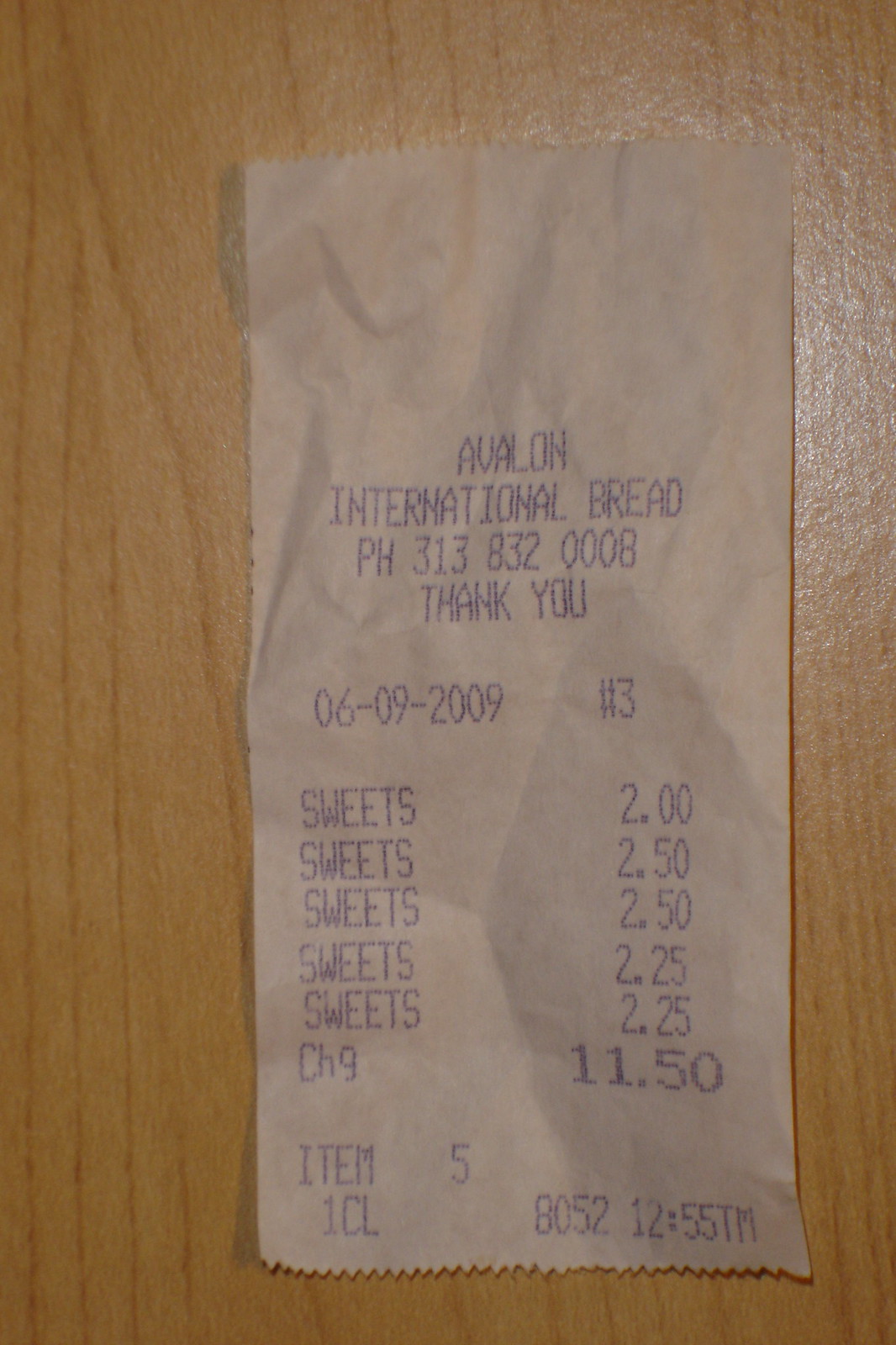A close-up image captures a crumpled white receipt from a purchase, suggesting it has been handled repeatedly. The receipt rests on a table with a whitewashed, light blonde wood finish. Printed in blue ink at the top of the paper, the receipt reads "Avalon International Bread," followed by the store's phone number and a polite "Thank you." The date, June 9th, 2009, is prominently displayed, detailing a transaction consisting exclusively of five entries labeled "sweets." The total amount for the purchases is $11.50, with the time of the transaction recorded as 12:55 PM.